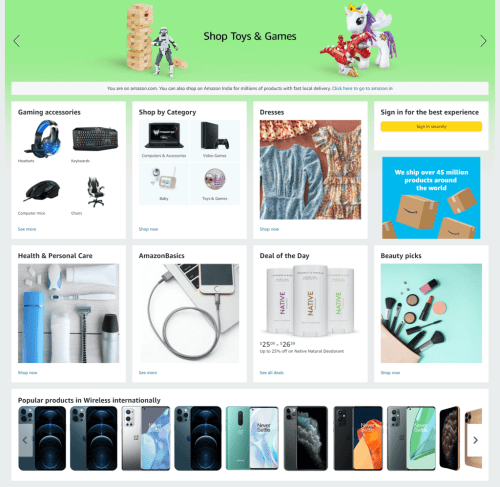The image features a prominent light green banner at the top with a less-than symbol (<) on the left and a greater-than symbol (>) on the right. In the center of this banner, there is an illustration of Jenga blocks, an action figure, and a unicorn doll with a purple mane, accompanied by the text "Shop Toys and Games."

Below this banner, the image becomes blurry, but several sections can still be made out. There is a box labeled "Gaming Accessories" showcasing a set of headphones, a mouse, a chair, and a keyboard. Adjacent to this, there is a "Shop by Category" section featuring a laptop and various other items.

Further down, another section displays images of a blue dress and a red dress under the label "Dresses." This is followed by a prompt that reads "Sign in for the Best Experience," accompanied by a large yellow button encouraging user login. 

At the bottom, a blue box contains images of cardboard boxes with some text above it. Below this, there is a "Beauty Picks" section featuring products like foundation, mascara, and makeup brushes.